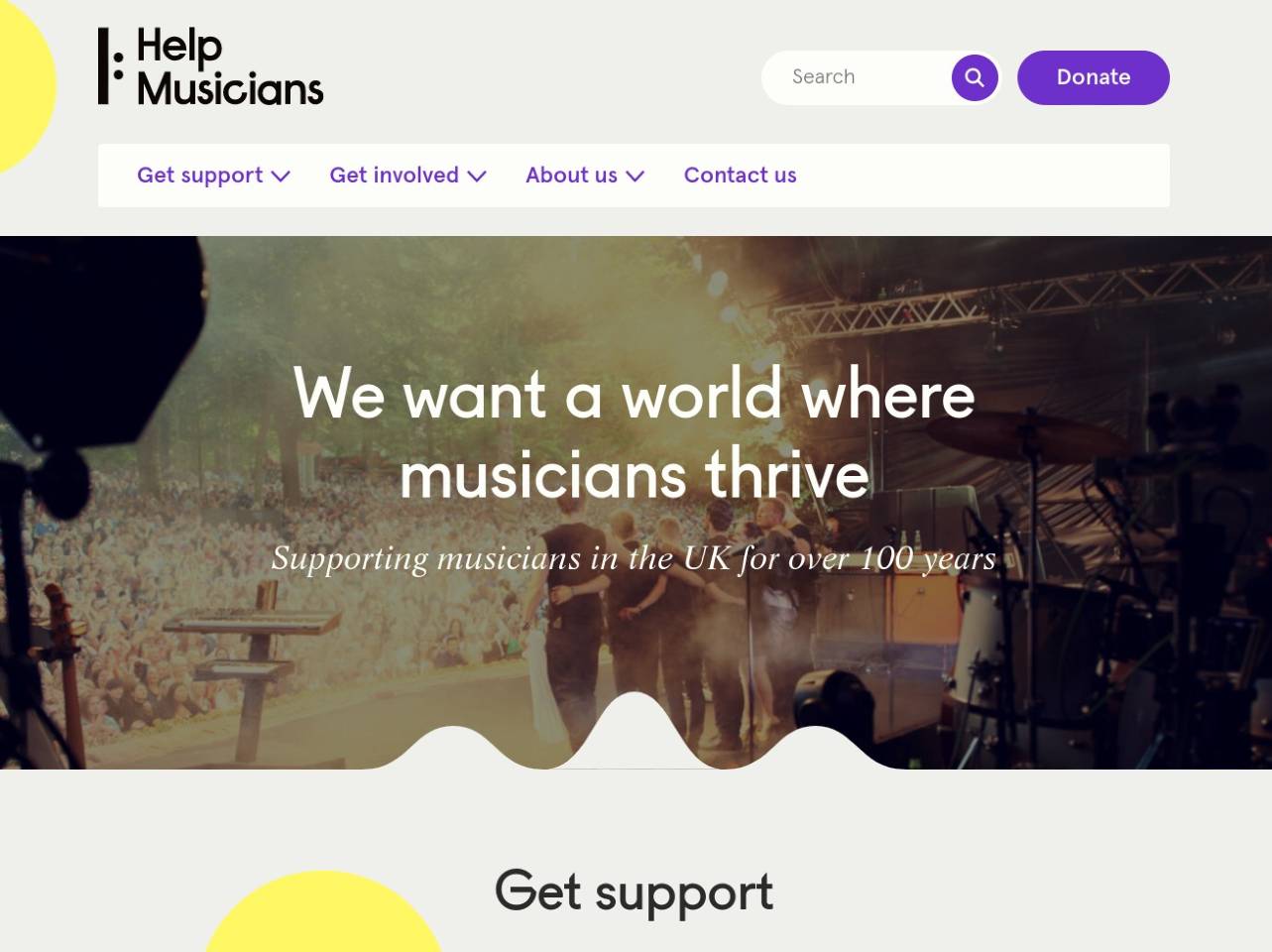The image depicts a website dedicated to supporting musicians. In the top left corner, bold black letters read, "Help Musicians," accompanied by a small sideways face icon and a half yellow circle emerging from the left side. On the right, there is a search bar featuring a purple circle with a white magnifying glass and next to it, a purple button labeled "Donate" in white text. Below is a navigation menu with drop-down options labeled, "Get Support," "Get Involved," "About Us," and "Contact Us."

Centered beneath the navigation menu is an image, seemingly of a music festival, overlaid with bold white text: "We want a world where musicians thrive. Supporting musicians in the UK for over a hundred years." The image extends down to a border of the same grayish-cream color found at the top.

Just below the image, bold black letters announce "Get Support." At the bottom, another half yellow circle appears, continuing the thematic design elements. The entire page emphasizes support for musicians in the UK.